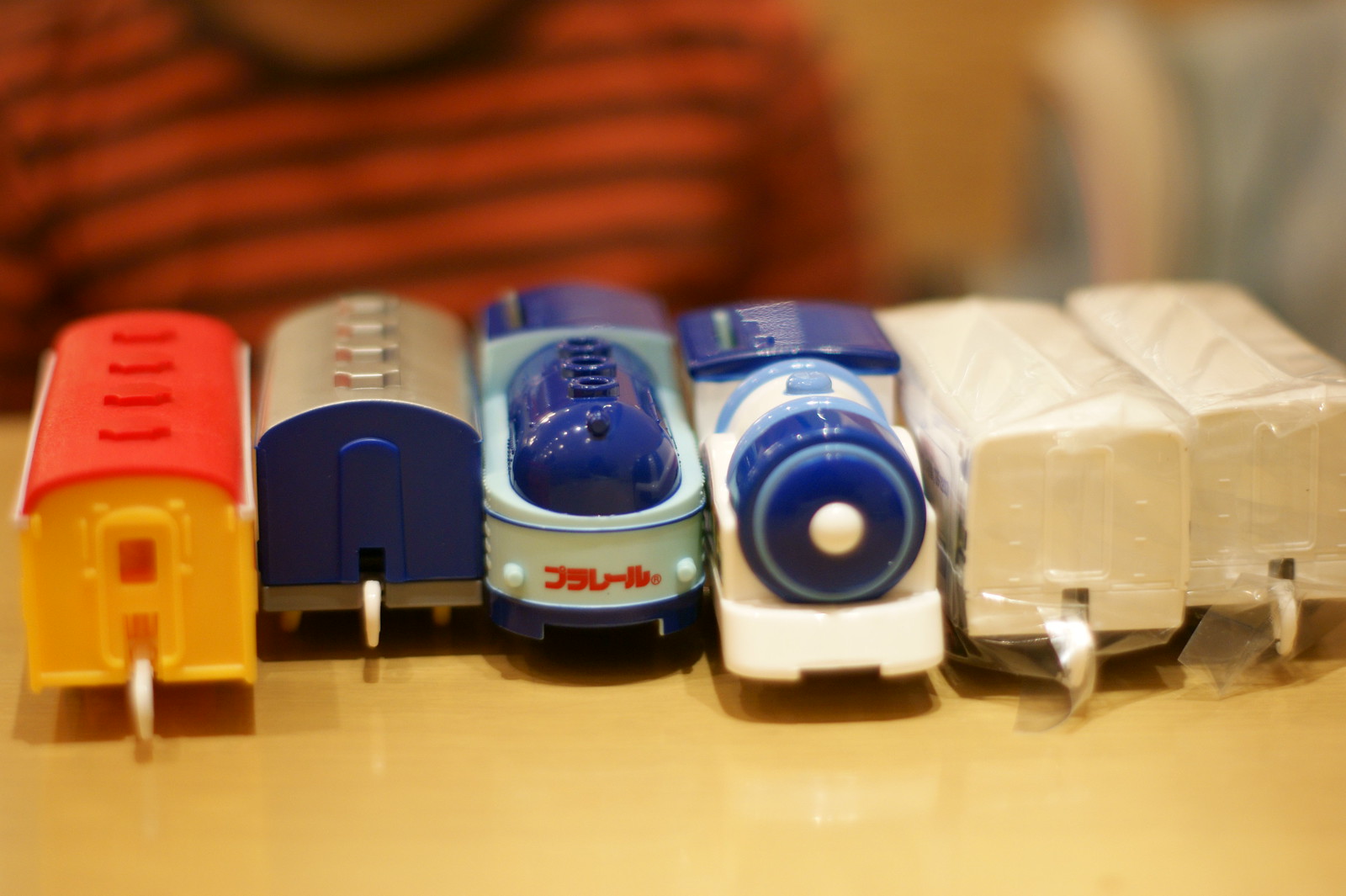In the foreground of the photograph, there is a colorful and detailed six-piece children's toy train set arranged neatly on a high-gloss, light tan brown wooden table. The train set comprises an engine and five box and passenger cars, featuring vibrant colors such as red, yellow, blue, orange, white, and silver. Each car is distinct, with the first car being dark yellow with an orange roof and a hook to connect to the next car. The second car is blue with a gold top, followed by a light and dark blue car with nondescript lettering, likely serving as the caboose. The fourth car is white with a blue top and rounded front, while the last two cars are light brown, potentially wrapped in plastic, indicating they are new or being preserved.

The train cars are positioned with their shorter ends facing towards the viewer, emphasizing their front hooks and details. In the background, slightly out of focus, is a child dressed in a red shirt with black horizontal stripes and a visible neck and chin, indicating anticipation to play with the train set. The child's head and lower body are out of the frame, emphasizing the focus on the toys.